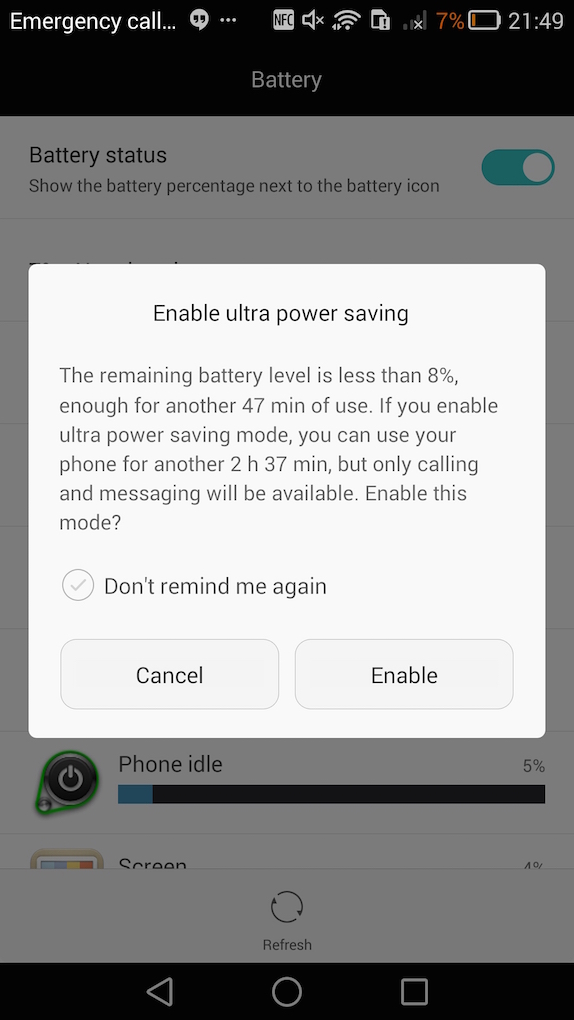The image captures a mobile device screen displaying a pop-up notification amid an interface characterized by several status indicators. 

At the topmost part of the screen, against a black background, a series of white icons and text are displayed. On the top left, "Emergency Call..." is visible, followed by a chat bubble logo containing two quotation marks. A series of system status icons follow: an NFC icon, a muted volume icon, a fully connected Wi-Fi indicator, an unfamiliar notification that might indicate an SD card issue, a signal strength icon showing no signal (depicted by empty bars with a white 'X'), and a red battery icon indicating 7% remaining battery life. The time, "21:49", is shown on the far right.

Directly below this status bar is the word "Battery," centered on the screen in a light grayish color, marking the end of the black background area and the beginning of the phone’s content area, overlaid by a pop-up notification related to battery status.

The underlying screen appears to be the phone's battery settings, partially obscured by the pop-up. The visible portion indicates "Battery status" with the option "Show the battery percentage next to the battery icon" enabled via a toggle switch, followed by a line break.

The prominent pop-up, slightly rounded at the corners, contains crucial information and options:
- A title: "Enable Ultra Power Saving"
- A paragraph warning that the battery level is less than 8%, estimating 47 minutes of remaining usage and offering an option to extend this to 2 hours and 37 minutes through Ultra Power Saving Mode, with a caveat that only calling and messaging will be available.
- An option labeled "Don't remind me again."
- Two buttons: "Cancel" on the left and "Enable" on the right.

Below this pop-up, the screen shows part of the battery settings interface. On the left, a power button icon with a green outline and next to it, a label "Phone idle" with a bar indicating usage: a small light blue segment (approximately 5-10%) and a larger dark blue segment, alongside a "5%" indicator on the right.

At the very bottom, a partially visible setting with the top half of the word "Screen" and a multicolored icon can be seen, along with a central "Refresh" icon and word at the screen's bottom center. The image concludes with the phone's navigation bar, featuring a left-pointing triangle, a circle, and a square on a black bar.

This detailed representation captures the user's mobile interface during a critical low-battery warning.